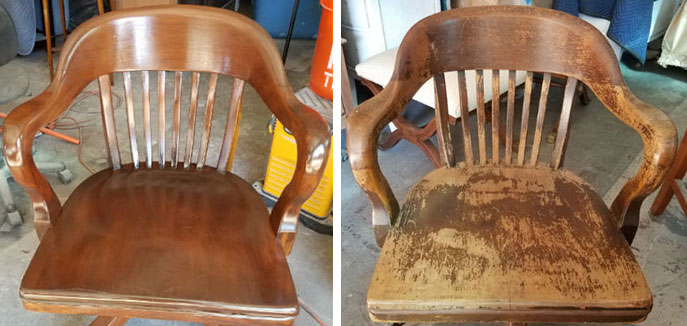The image features a side-by-side comparison of a wooden chair before and after it has been refinished. Both pictures are taken in a workshop with a concrete floor and a nondescript background. The chair has a rounded back and partial armrests with eight vertical columns supporting the backrest. In the right-hand picture, the chair appears heavily worn and scratched, showing significant wear on the seat and armrests, with the finish almost completely worn off, revealing the bare wood. In contrast, the left-hand picture showcases the same chair after it has been meticulously refinished. The restored chair boasts a shiny, dark brown hue with a polished, inviting appearance, free of scratches and blemishes. This detailed juxtaposition highlights the transformation achieved through the refinishing process.